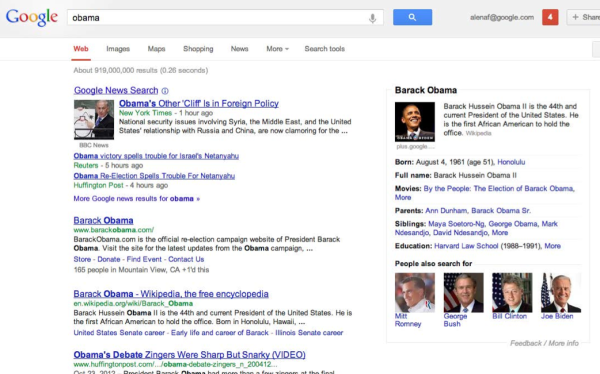This image is a screenshot of a Google search results page. At the top left corner, the Google logo is prominently displayed. The search bar contains the query "Obama," with the blue search icon visible to its right. Below the search bar, several tabs provide filtering options: "Web," "Images," "Maps," "Shopping," "News," "More," and "Search tools."

The top search result is from Google News: "Obama's other cliff is in Foreign Policy." Following this, news headlines mention "Obama Victory," "Tribute for Israel's Netanyahu," and "Obama Re-Election Spells Trouble for Netanyahu." The next listing is from barackobama.com, labeled as the official re-election campaign website for President Barack Obama, inviting visitors to explore for updates.

Further down, the Wikipedia entry for Barack Obama appears, introducing him as the 44th and current President of the United States and the first African American to hold the office. It briefly touches on his birthplace—Honolulu, Hawaii.

A video result titled "Obama's debate zingers were sharp, but snarky" is also listed.

On the right side of the screen, a sidebar provides a concise profile of Barack Obama, including a photograph. It reiterates his position as the 44th President, born on August 4, 1961, age 51, in Honolulu, and lists some of his notable works, such as the movie "By the People: The Election of Barack Obama." Additionally, it features a section titled "People also search for," which includes Mitt Romney, George Bush, Bill Clinton, and Joe Biden.